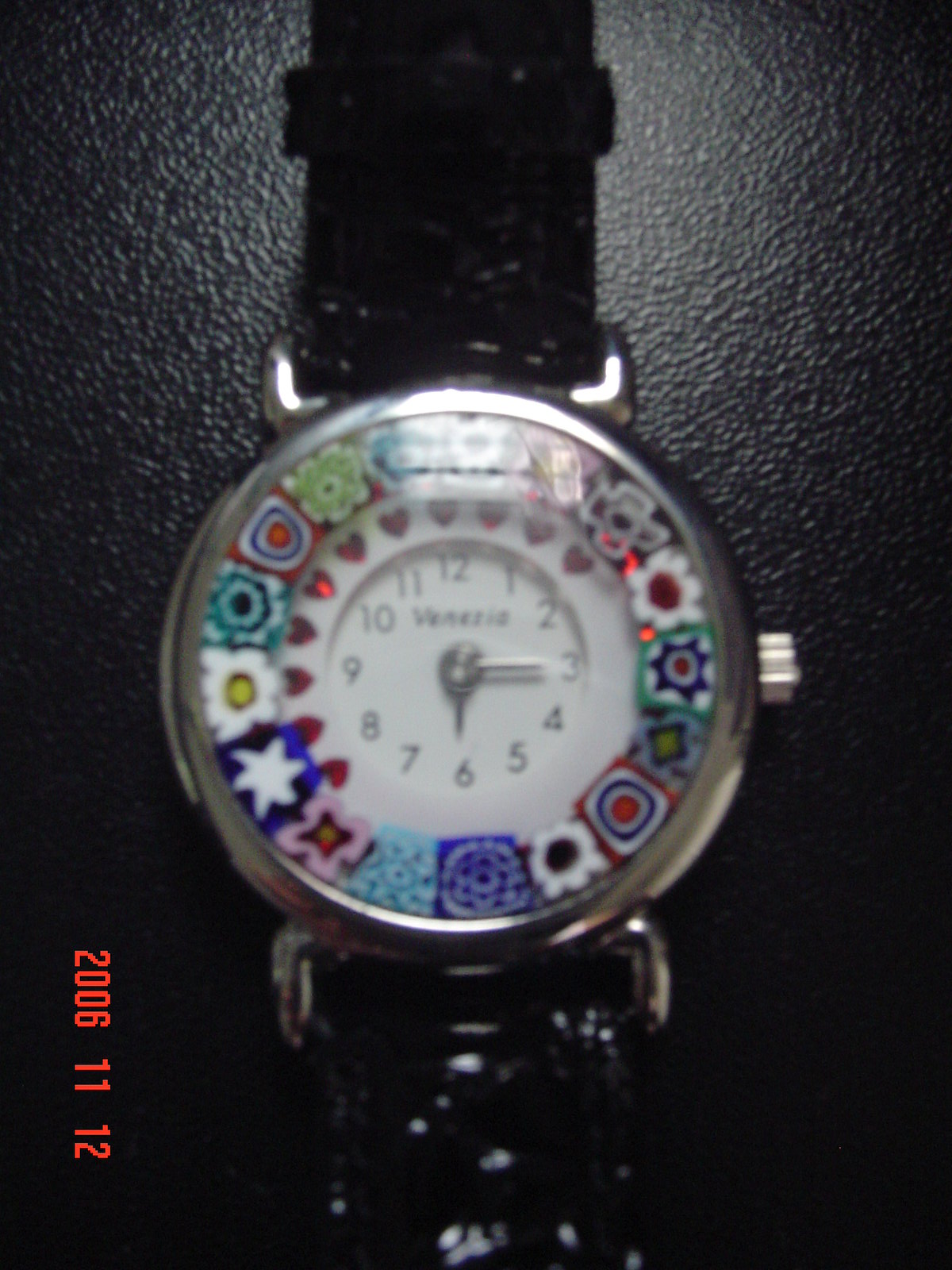This up-close photograph showcases a Ritz watch resting on a sleek, black, leather-like surface. The watchband, only partially visible at both the top and the bottom of the frame, appears to be black with a slightly slippery, wet sheen, and features silver clasps. The watch itself is positioned centrally and highlighted by a surrounding silver bezel, with a small, silver winding knob located on the right side.

The watch face is layered with intricate details. Around the outer rim, there appears to be a series of diverse designs including black, white, and blue star-like patterns and various shapes, all arranged in individual segments resembling squares. Unfortunately, a glare from a light obscures the top portion of the watch glass, masking some of these details.

Inside this decorative border, there is a prominent white ring adorned with red heart motifs extending from around the 2 o'clock to the 8 o'clock positions. This encircles the main dial, which features black numerals from 12 through to 12 in a clockwise fashion. There is also an inscription or lettering stretching from beneath the 11 to the 1 position, although it is too indistinct to read. 

At the very center, the dial includes a small silver circle from which three silver hands emanate: the longer one pointing to the 3, another towards the 6, and the third hand extending to various other positions to display the time. The overall presentation combines precision with artistic detail, underlining the watch's elegant design and craftsmanship.